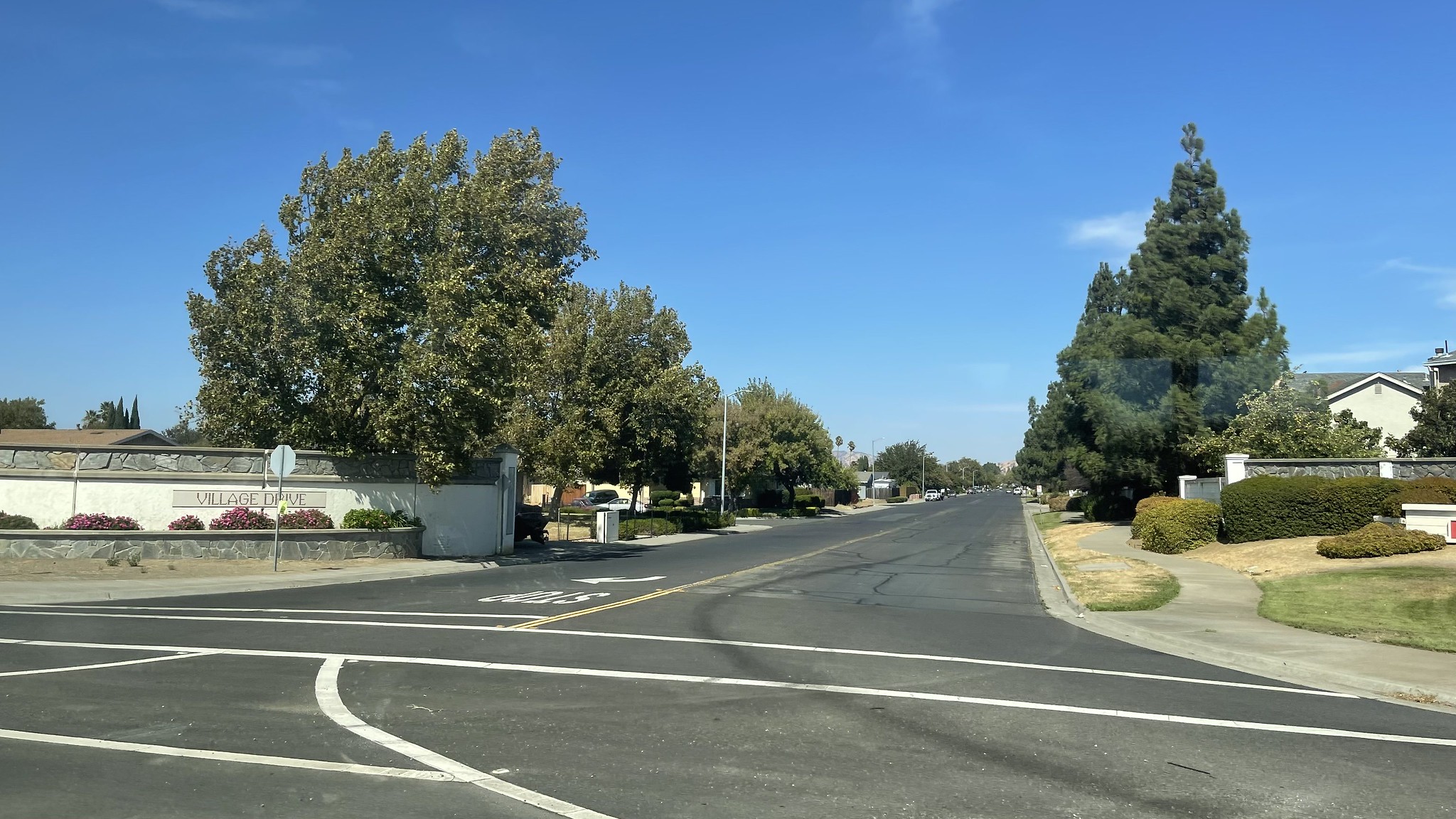This daytime color photograph captures a residential intersection reminiscent of a Google Street View snapshot. Taken from a standing height in the middle of the intersection, the image affords a broad view of the area. The intersection is marked with prominent white painted lines, including the word "STOP" accompanied by a right-turn arrow clearly visible on the asphalt. The sky above is a vivid blue, dotted with just a few sparse clouds, emphasizing the bright, sunny weather.

Surrounding the intersection are a few two-story homes, which appear to be in the ranch style. These homes are complemented by patches of grass that vary from faded tan to a deep green, indicating areas of dying and thriving vegetation. Trees are sporadically placed, adding some greenery to the suburban setting. 

A stop sign is notably present, though only its backside is visible in the photograph. Additionally, a white wall prominently displays a nameplate reading "Village Drive," signaling the entrance to the residential neighborhood. This nameplate is enhanced by modest landscaping and hardscaping features.

The street is notably tranquil, with no vehicles in the immediate vicinity. However, one or two cars can be seen parked far down the street along the curb, reinforcing the calm and serene environment of the neighborhood.